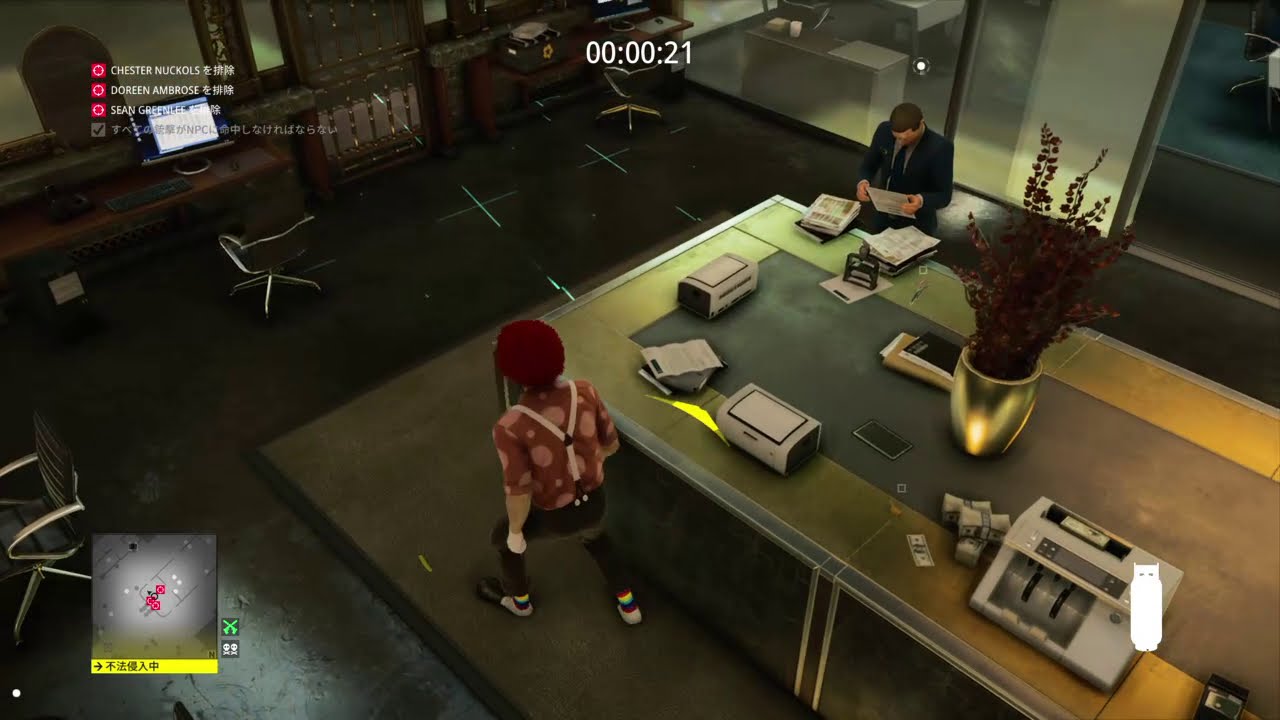This screenshot from a video game presents a third-person view of a dimly lit corporate office filled with high-tech gadgets and office equipment. At the center of the scene, a character stands out, wearing a dark maroon-colored hat, a brown shirt with pink spots, white suspenders, black pants, and gray and black shoes with green rings around the ankles. His left hand, either gloved or pale, hangs straight down. Beside him, on the right, is a large table cluttered with printers and electronic devices, and an open piece of paper near his shoulder. To the left of this character is a man in a black suit with a gray shirt and black tie, focused on some papers in his hands.

The upper left corner of the screen shows three pink squares with white circles, each displaying a name: Chester Nichols, Doreen Ambrose, and a partially obscured Sean. Above, in the center, there is a timer reading "00:00:21." A computer screen with a white document is visible in the background, blurred alongside tables with silver bottoms. 

In the far lower left corner, there's a partial view of a chair with a black backrest and silver armrests. The mini-map in the bottom left shows a gray interior with a yellow bar across the bottom featuring foreign characters. Meanwhile, the bottom right corner contains an emblem of a white owl.